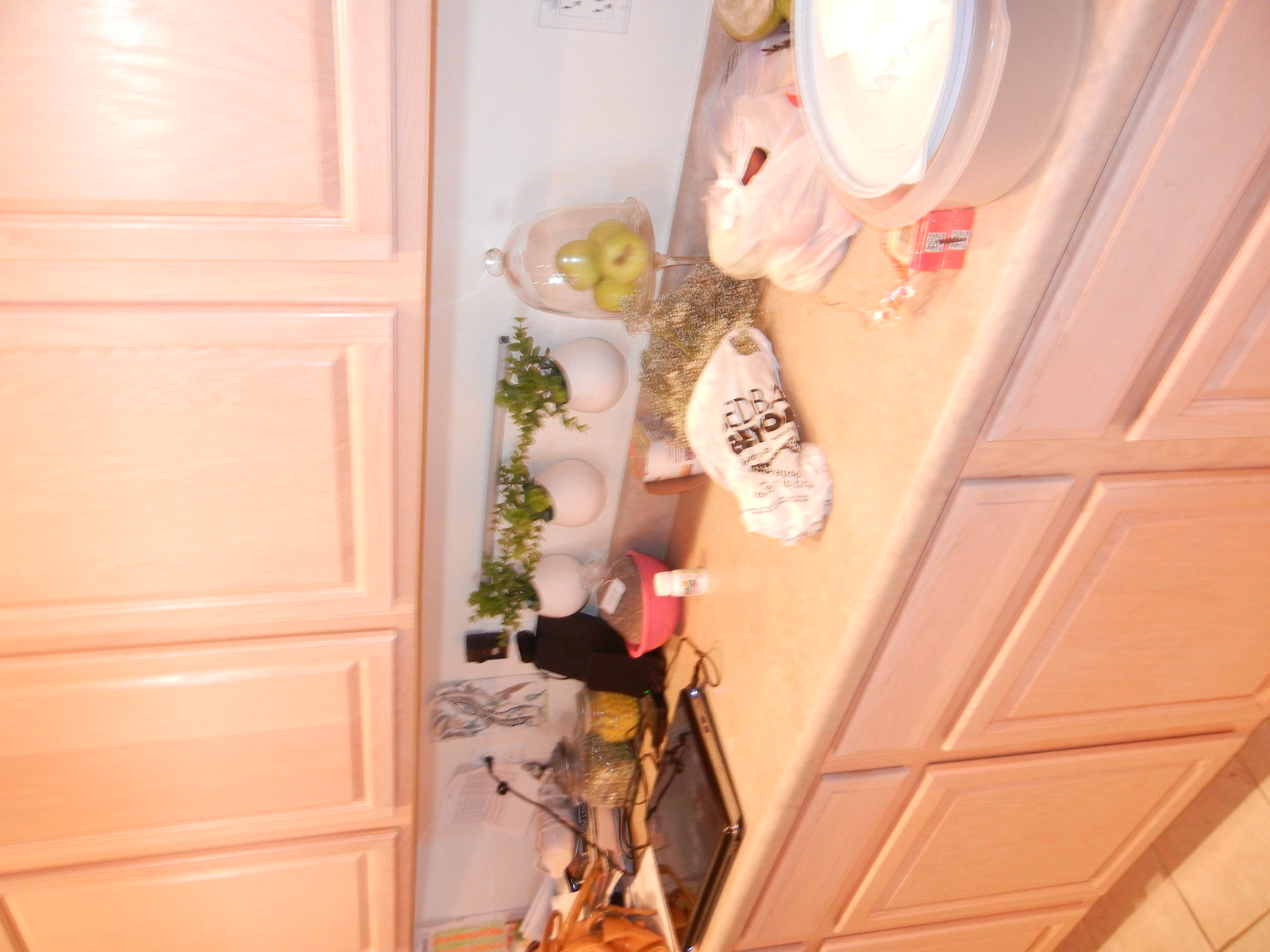The image depicts a kitchen counter captured from a sideways angle, with both upper cupboards and lower drawers visible, all sharing a light pink hue. On the countertop, a white plastic bag with black lettering takes the center position. To its right, a white plastic bag containing an assortment of apples or similar fruits is tied up securely. Adjacent to the fruit bag, a round plastic container featuring a light pink base and a white top can be seen. Further along the counter’s edge, a phone or tablet rests delicately. The wall beneath the upper cupboards is also visible, painted white and equipped with an electrical outlet on the right side. Above the counter, there are four cupboard doors, mirrored by four matching cabinet doors below. The floor tiles, exhibiting a squirt-like pattern, are partially visible and share the same light pink color scheme as the rest of the kitchen elements.